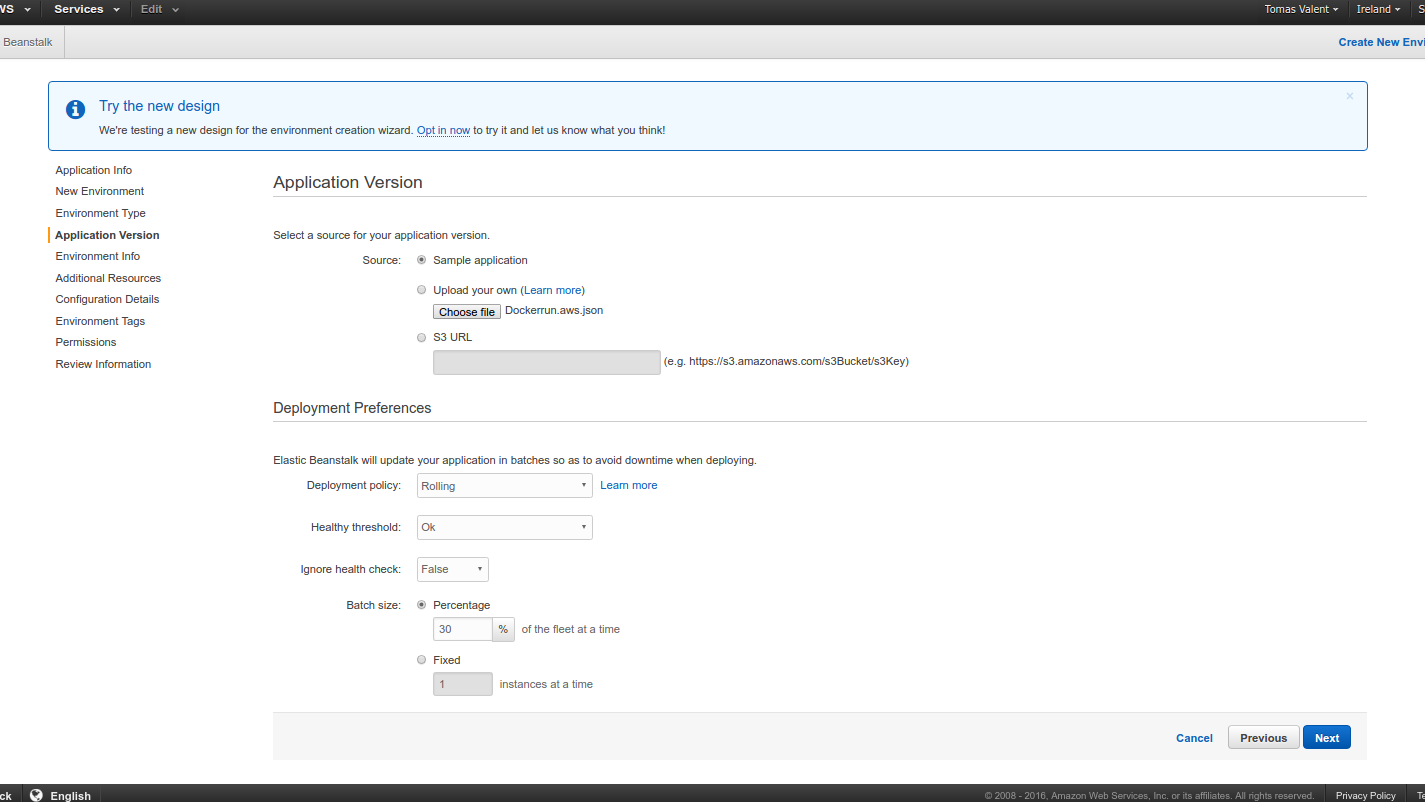The screenshot appears to be taken from a computer interface, possibly of a cloud service management console, involving deployment settings. 

At the very top, there's a black bar partially cut off, showing menu options: "VS," "Services," and "Edit," each with a drop-down menu. On the right side of this bar, there are user-specific options: "Thomas Valerick," a drop-down selection for "Ireland," and another cut-off menu labeled "S."

Beneath this, a prominent blue bar is labeled "Beanstalk." To the right of this bar, we can see an option for "Create New" and a truncated "ENV."

Below the blue bar, there is a narrower blue strip stretching approximately half an inch deep and eight inches wide, containing text prompting users to “Try the new design.” It invites users to opt into the new design for the "Environment Creation Wizard" and share their feedback.

In the main section, a vertical menu is visible on the left side, listing: "Application Info," "New Environment," "Environment Type," "Application Version" (highlighted in bold, indicating the current selection), "Environment Info," "Additional Resources," "Configuration Details," "Environment Tags," "Permissions," and "Review Information."

The main content pane is set to the "Application Version" page of the drop-down menu, showcasing various deployment options. Users can select a source for their application version, including options like "Source," "Sample Application," "Upload Your Own," and "S3 URL."

Deployment preferences are detailed next, indicating that "Elastic Beanstalk" will update the application in batches to prevent downtime. Users can adjust the "Deployment Policy" to "Rolling" and set the "Healthy Threshold," with options for "OK" or "Ignore Health Check." The "Batch Size Percentage" is set at 30%, though another option could be "fixed one instance at a time."

This screenshot provides an overview of the deployment settings page within the "Beanstalk" environment, emphasizing user controls and deployment configurations.